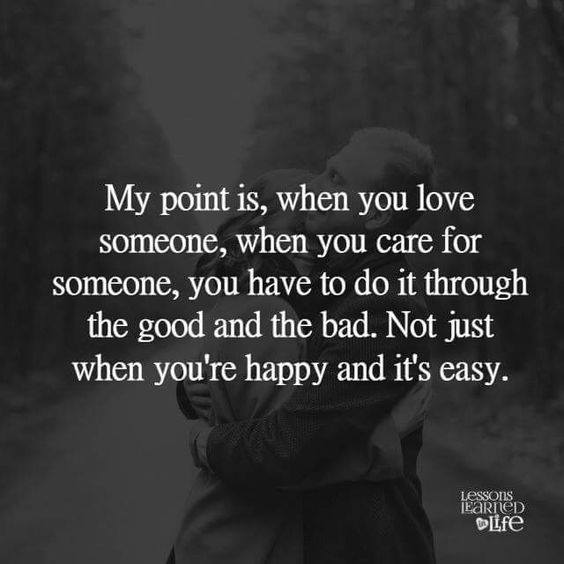The image is a square, black-and-white photograph, featuring a man and a woman standing on a rural road, surrounded by trees on both sides. The man, who is taller, stands on the right and embraces the woman, his eyes closed and a slight smile on his face. Both are wearing dark coats, and the scene is set against a backdrop of a clear sky framed in a V-shape by distant hills. The photograph is faded and overlaid with a semi-transparent gray filter to highlight the text. The quote, written in a Times Roman-like font in mixed upper and lower case, reads: "my point is, when you love someone, when you care for someone, you have to do it through the good and the bad, not just when you're happy and it's easy." In the bottom right corner, in bold white letters, it says "LESSONS LEARNED" followed by a small heart icon containing the word "life."